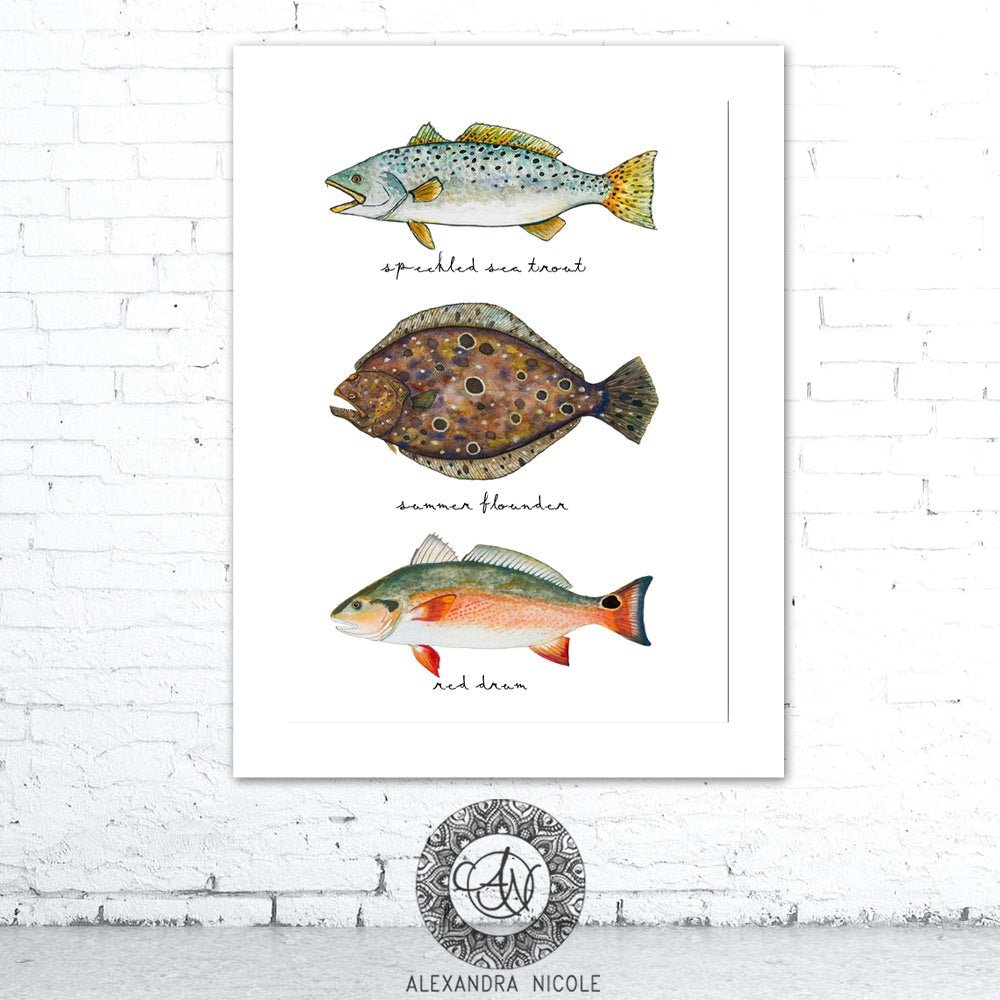The image is a detailed product photograph of a poster print featuring three fish, each depicted in a painted style and oriented vertically with their mouths open to the left. The artwork is displayed against a white brick wall, and the floor below is gray concrete. The poster is framed in white. 

At the top of the poster is a speckled sea trout, characterized by its silver body adorned with black dots and yellow fins. Its name, "speckled sea trout," is written in cursive beneath it. The middle fish is a summer flounder, with a flat brown body marked by numerous brown circles. Its name, "summer flounder," also appears in cursive beneath it. The bottom fish is a red drum, featuring a gray upper body transitioning into a red lower body, with a distinctive black spot on its tail. "Red drum" is inscribed in cursive below this fish.

At the bottom of the poster is a logo consisting of an elaborate geometric circle enclosing the initials "A-N" in script, followed by the name "Alexandra Nicole."